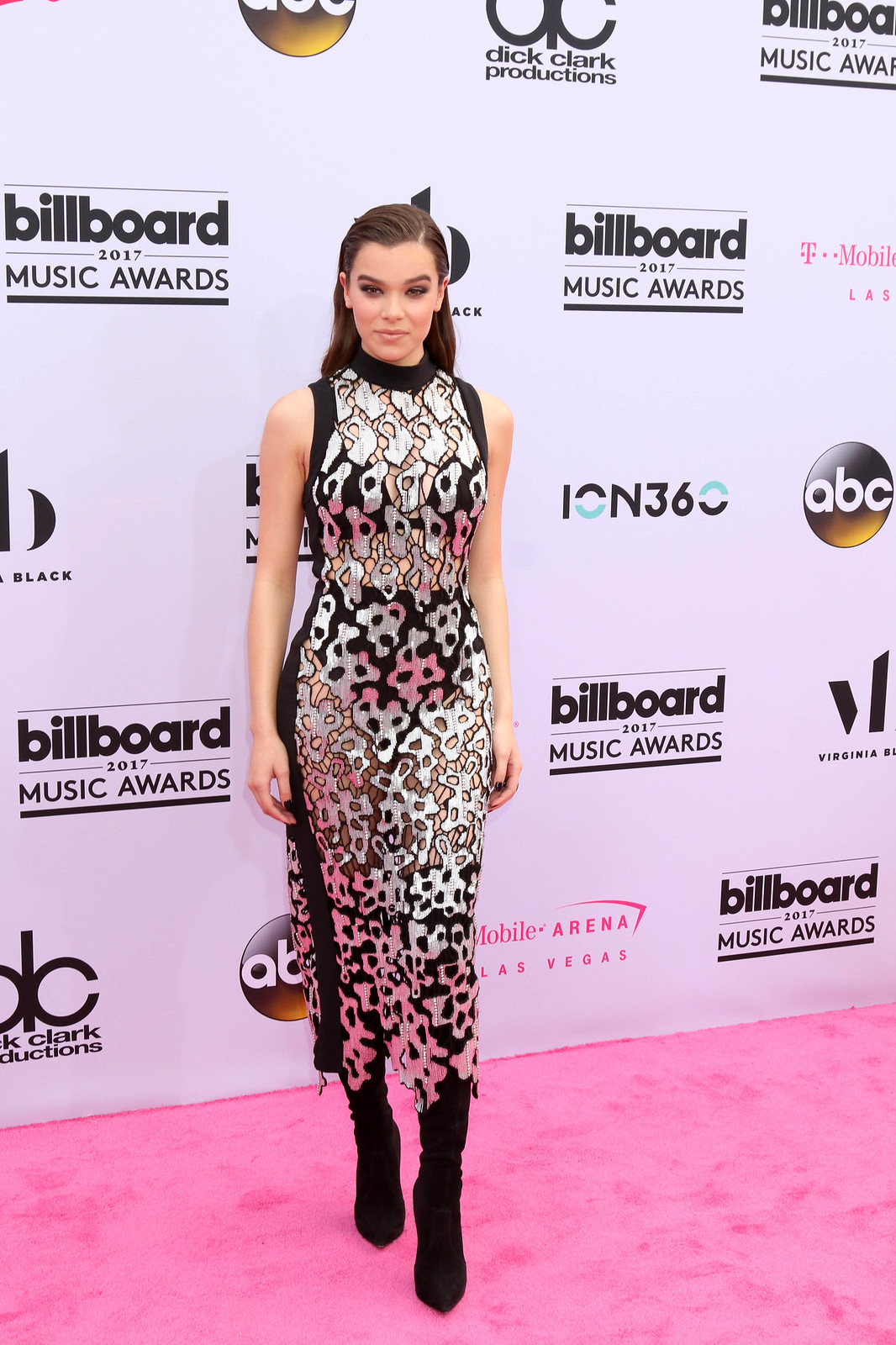Haley Steinfeld is seen posing on a pink carpet at the Billboard Music Awards 2017. The backdrop behind her features a repeating pattern of logos and text, including "Billboard 2017 Music Awards," "ABC," "T-Mobile," "ION 360," "Mobile," "Arena," and "Las Vegas." Haley is wearing a sleeveless long dress with a striking print in black, white, yellow, and pink, complemented by black boots. Her long, dark hair is parted on the right-hand side and slicked back. The entire setting mimics a red carpet event but uniquely uses a pink carpet.